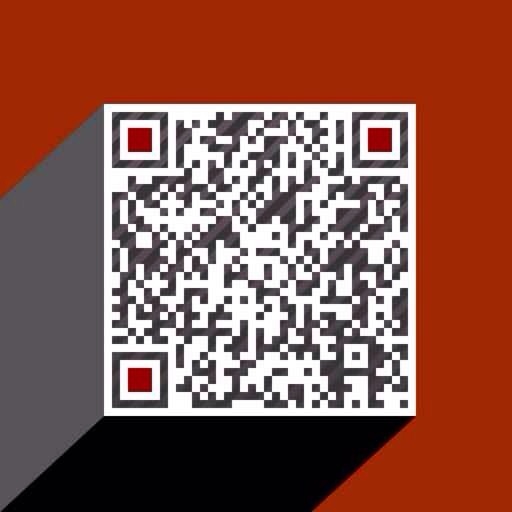The image is a computer-generated square with a dominant light red background. Emerging from the left side is a three-dimensional cube, showing three visible faces. The cube's left face is gray, the bottom face is black, and the front face displays an intricate QR code, characterized by its typical black and white pattern. Each corner of the QR code—top left, top right, and bottom left—features a smaller red square bordered by alternating black and gray stripes. The QR code stands centrally, occupying most of the image space, and is free from any additional text or embellishments. The intersecting lines within the QR code, alongside the red, black, and gray elements, create a visually striking composition.